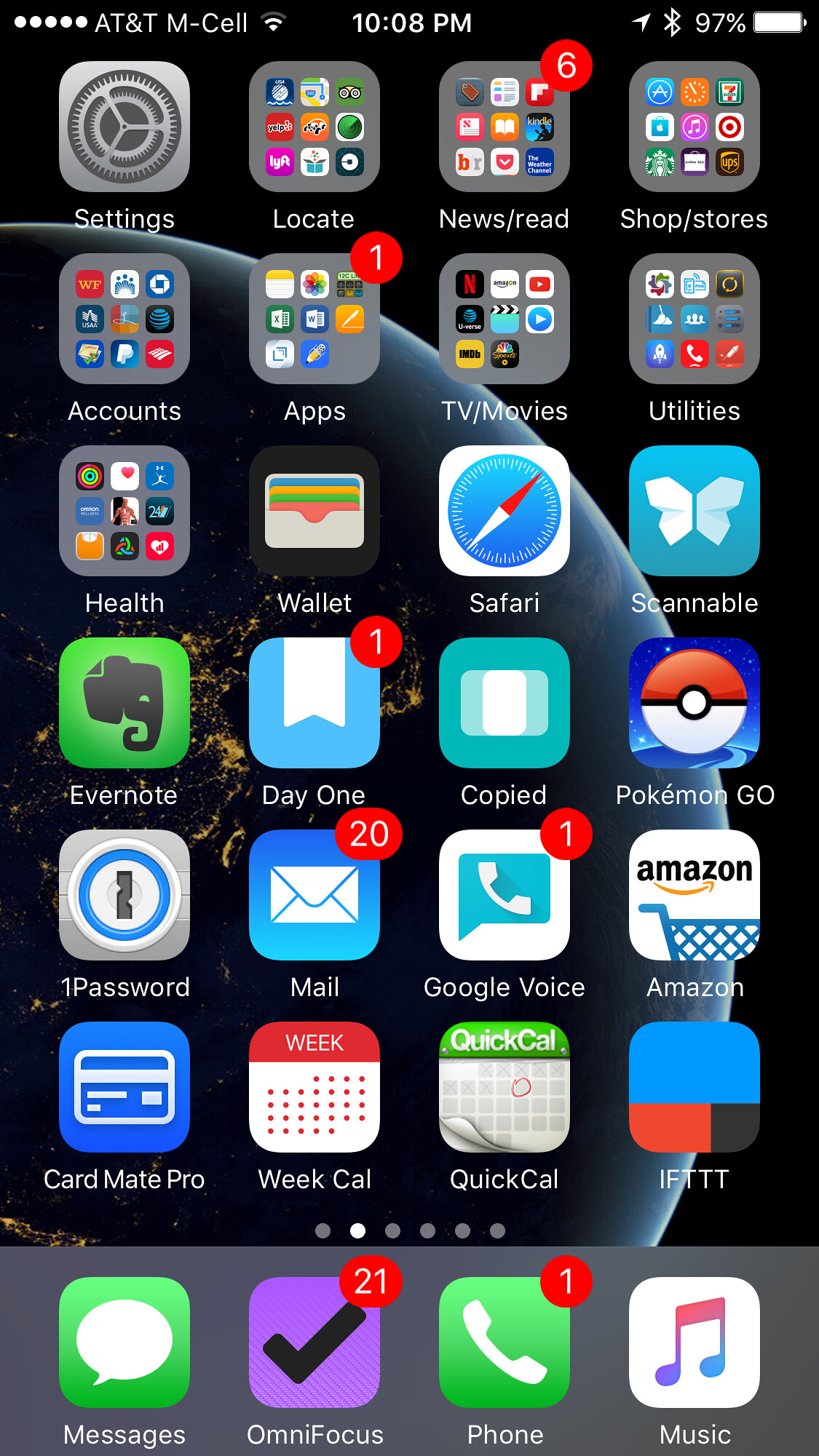In the image, we see a typical smartphone interface against a black background that appears to depict a planet illuminated by city lights at night. At the top of the screen, from left to right, there are indicators and icons as follows: five white dots indicating cellular signal strength, the "AT&T M-cell" network label, a Wi-Fi signal icon, the time reading "10:08 PM," and a battery icon indicating a 97% charge with a fully white battery shape.

Beneath this status bar, the home screen is organized into several rows of app icons and folders. The first row features settings, locate, news/read, shop, and stores folders, each represented by small, grey square icons. The next row includes a red circle with the number six beside the news/read folder, accounts, apps with a red circle indicating one notification, TV, movies, and utilities.

Continuing downward, the subsequent rows host various applications: health, wallet, safari, scannable; Evernote with its green elephant logo, day one with a red circle and number one, copied, and Pokémon Go. Further down, we see one password, mail with a red notification circle indicating 20 unread items, Google Voice with a red circle showing one notification, and Amazon.

The last few rows consist of CardMate Pro, WeCall, QuickCall, and IFTTT. At the bottom of the display, there are six navigation dots, with the second dot from the left filled white, indicating the current home screen page. The final row on a grey background contains messages, OmniFocus with a red circle showing 21 notifications, the phone app with a red circle indicating one missed call, and music.